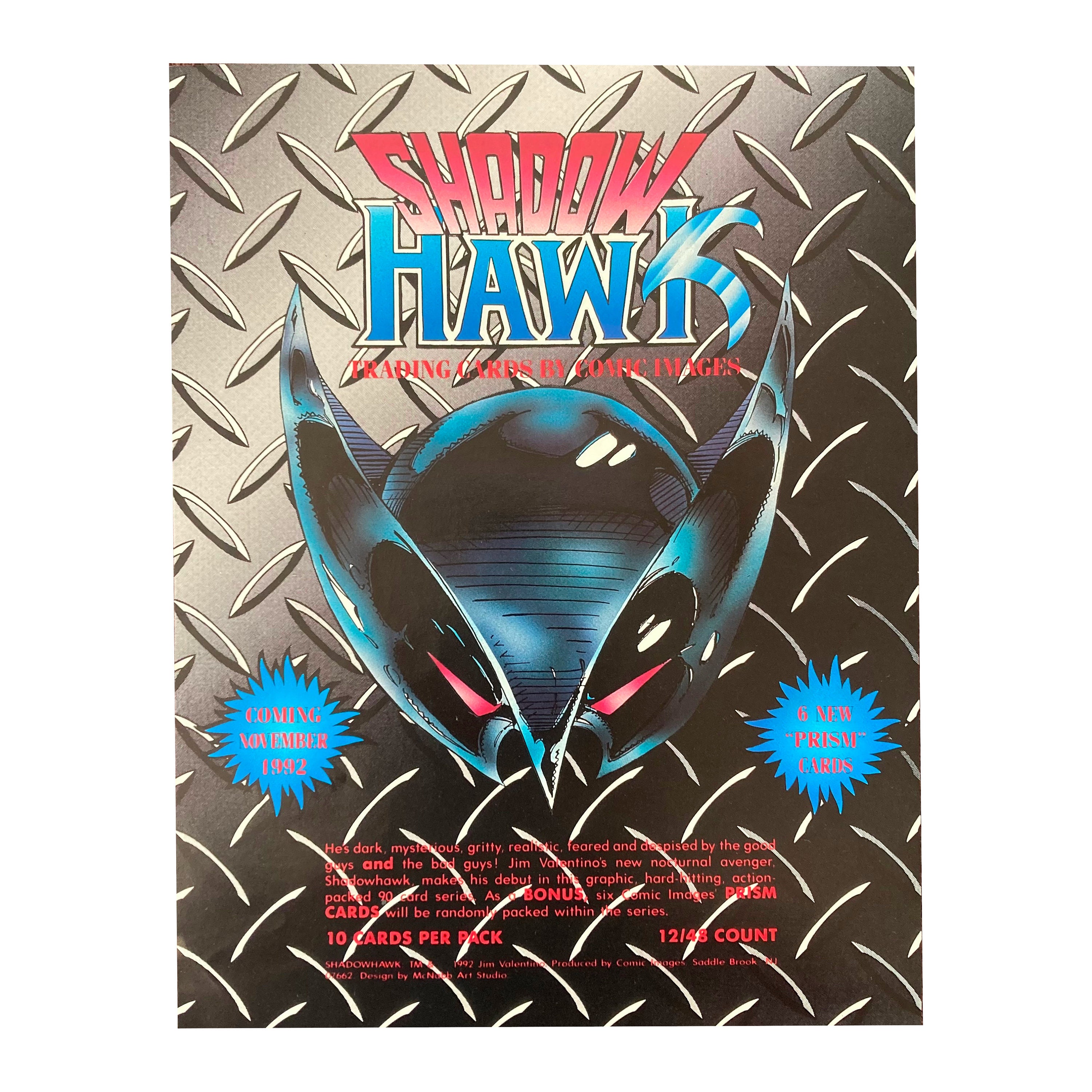The image depicts a promotional poster for Shadowhawk Trading Cards by Comic Images. The background features a metal grid pattern, adding a dynamic and gritty texture to the overall design. Prominently displayed at the top of the poster, white text announces the title, "Shadowhawk Trading Cards by Comic Images." Beneath this is a striking helmet or mask, characterized by red triangular eyes and flaring sides resembling ears, designed to cover the upper part of the head. Below the helmet, in bold red text, the poster teases the upcoming release: "Coming November 1992." It further describes Shadowhawk as dark, mysterious, gritty, realistic, feared, and despised by both good and bad characters. The text highlights the creator, Jim Valentino's dark, nocturnal Avenger, Shadowhawk, making his debut in a hard-hitting, action-packed 90-card series. An additional note mentions that the new Prism Cards will be included, promising six new designs randomly packed within the series, with 10 cards per pack and 12/45 count packs. The dominant colors of the poster are black and red, enhancing its bold and intense visual appeal.